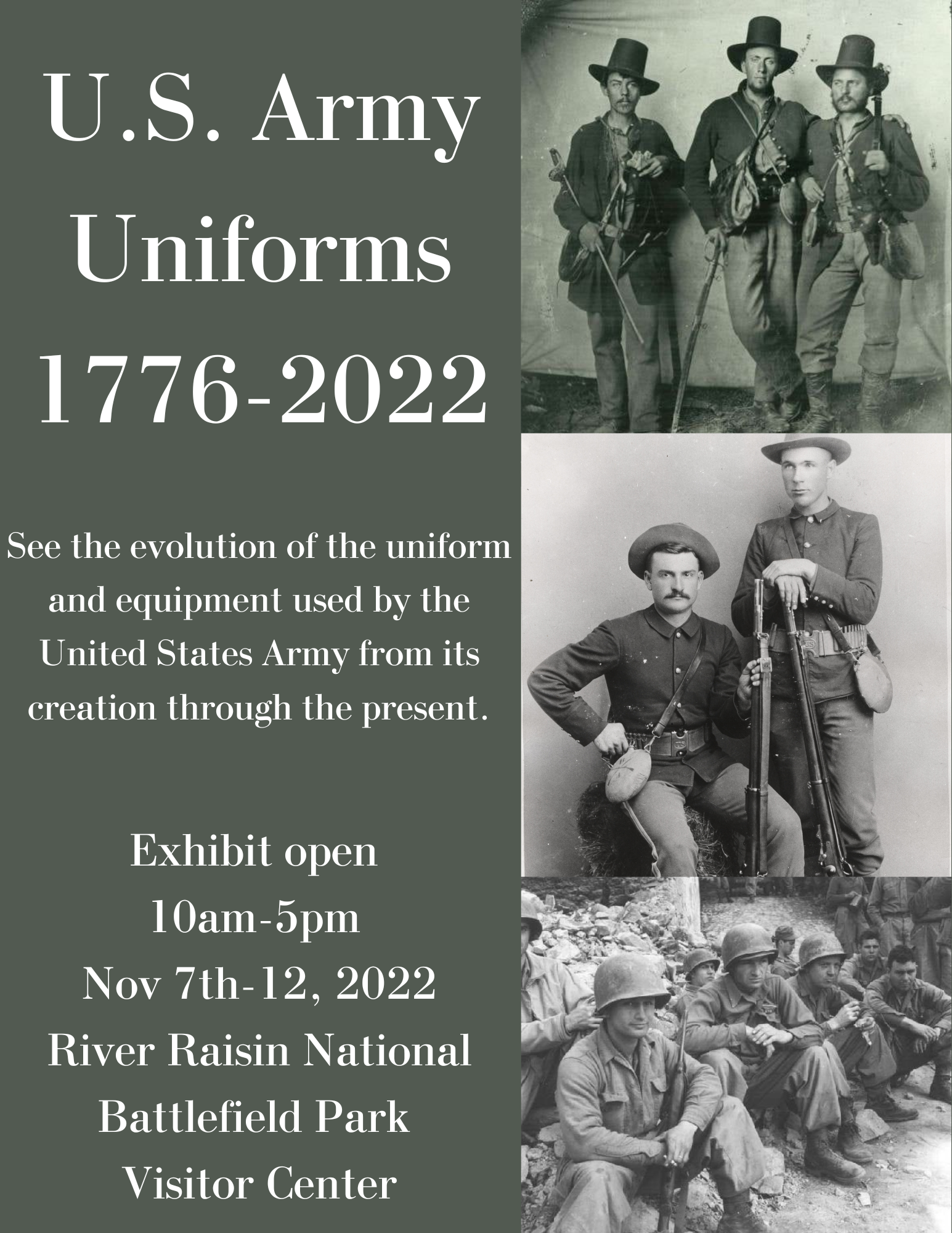A detailed black and white poster promoting a museum exhibit features a left-hand column of white text set against a dark green background, reading: "U.S. Army Uniforms, 1776-2022. See the evolution of the uniform and equipment used by the United States Army from its creation through the present. Exhibit open 10 a.m. to 5 p.m., November 7-12, 2022, River Raisin National Battlefield Park Visitor Center." On the right-hand side, arranged vertically, are three black and white photographs of soldiers in uniform from different eras. The top image likely depicts a soldier from the Revolutionary War, the middle image shows a Civil War soldier, and the bottom image features a World War II-era soldier. Each photograph captures the soldiers in period-specific uniforms, highlighting the historical changes.